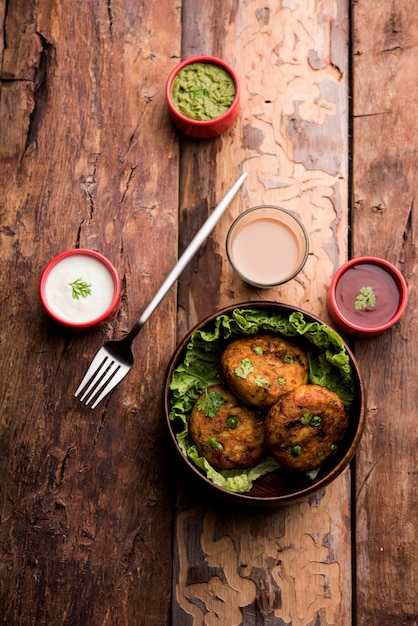This is an overhead photograph of a beautifully arranged table setting, showcasing a variety of foods and condiments on a rough-hewn wooden table. Central to the image is a round bowl containing three browned, circular patties, possibly chickpea fritters or another type of dumpling, resting on a bed of large, open lettuce leaves. These patties are garnished with chopped parsley and green onions. Surrounding the central bowl are four smaller containers of dipping sauces: a white sauce with dill located to the left, a whitish-red mayonnaise-based sauce in the center, and a red sauce to the far right. Additionally, there is a small red bowl at the top containing a green ingredient, potentially mashed avocado or guacamole. To the side of the sauces, a long-handled silver fork lies on the table. The rustic wood of the table adds a charming, earthy backdrop to the colorful and well-presented food.